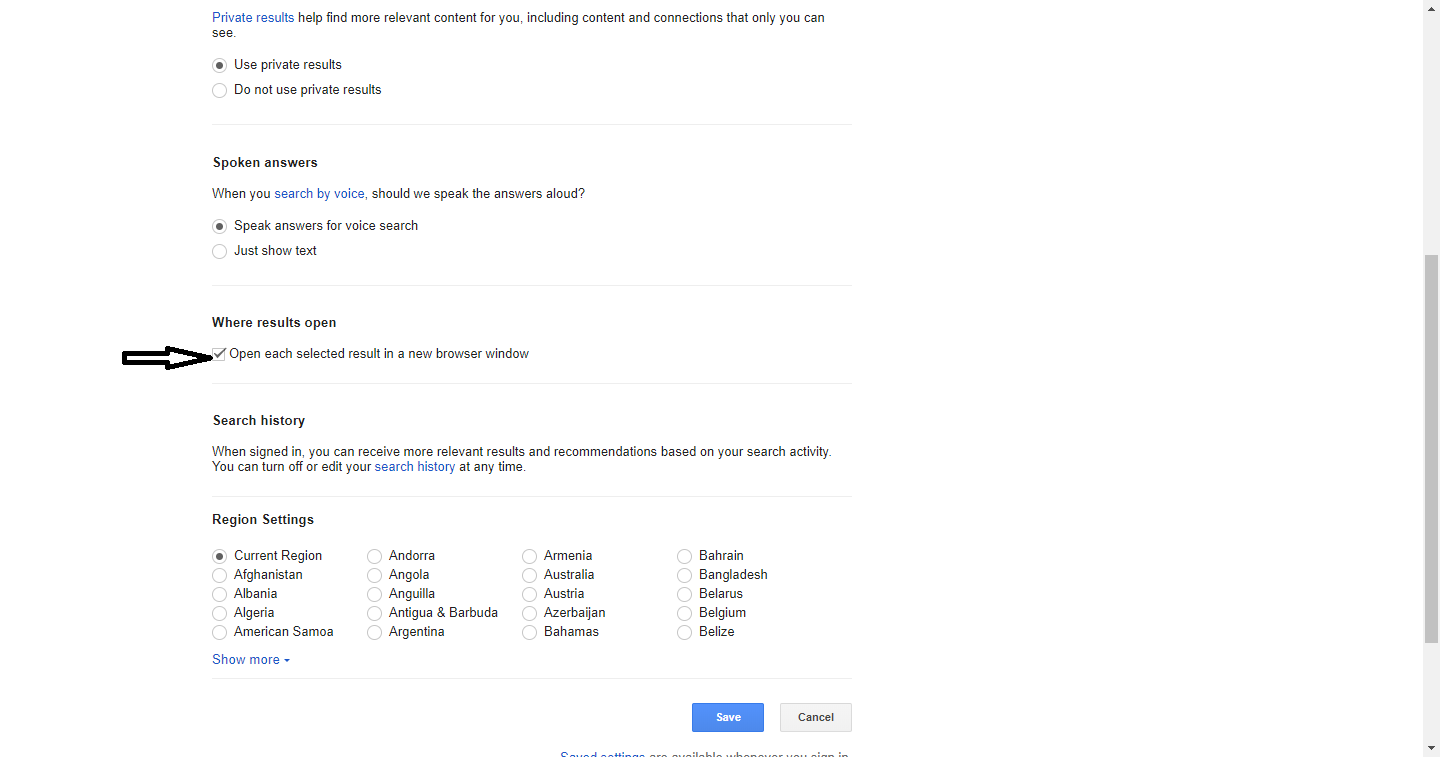The image depicts a user interface screen displaying various search settings options. At the top, there's an option labeled "Private results" which allows users to enable or disable finding more relevant content through personalized connections; it is currently set to "private results." Below this, a section labeled "Spoken answers" features a highlighted option for "Search by voice" in blue, asking whether search answers should be spoken aloud or just shown as text. 

Further down, there is a "Where results open" checkbox which is selected, indicating that each selected result will open in a new browser window. A long hand-drawn arrow points to the left of this feature for emphasis. 

"Search history" is the next section, informing users that signing in enables receiving more relevant results and recommendations based on past search activity. Users can also edit or turn off their search history anytime. 

"Region settings" lists the current region and offers a dropdown menu to select other countries alphabetically from Afghanistan to Albania, with an option to "show more" regions. 

At the bottom right, there are two buttons: a blue "Save" button and a "Cancel" button. The interface background is white, keeping the design simple. Additionally, key options such as "Private results," "Search by voice," and "Show more" are displayed in blue, while the "Save settings" feature appears to be slightly cut off at the bottom of the image.